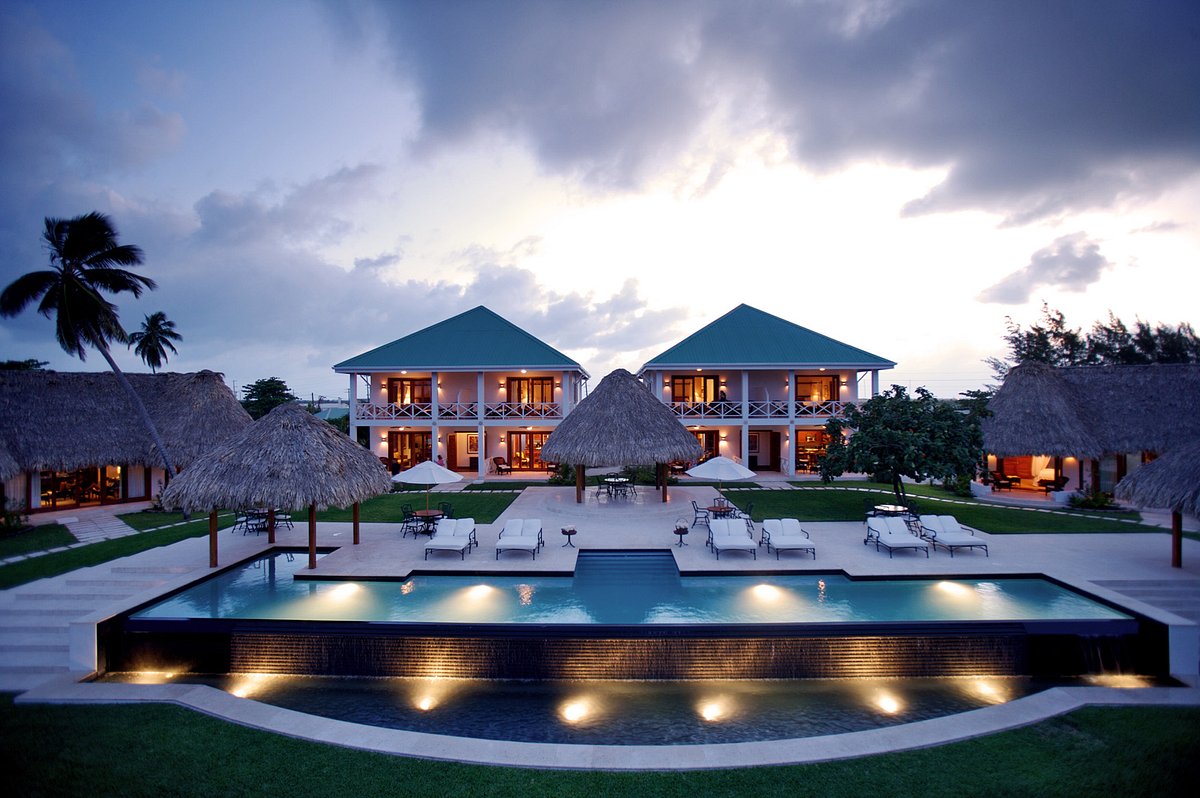The image depicts a serene resort at dusk, bathed in soft lighting. Dominating the foreground is a rectangular pool framed with lounge chairs and festive lights shimmering on its sides. Flanking the pool are two symmetrical, two-story buildings, their interiors warmly illuminated against the growing darkness. These buildings feature cyan-blue, triangular, wooden roofs. Nestled centrally between them is a charming conical-roofed hut with open walls, contributing to the ambient resort atmosphere.

On either side, smaller cabins with thatched-style leaf rooftops add a rustic touch to the scene. Palm trees stand gracefully on the left, while a neatly manicured lawn stretches out in the center. The sky above is a blend of remnant light and darkening clouds, hinting at the recent sunset. The overall vibe of the resort is tranquil and inviting, perfect for a relaxing getaway.